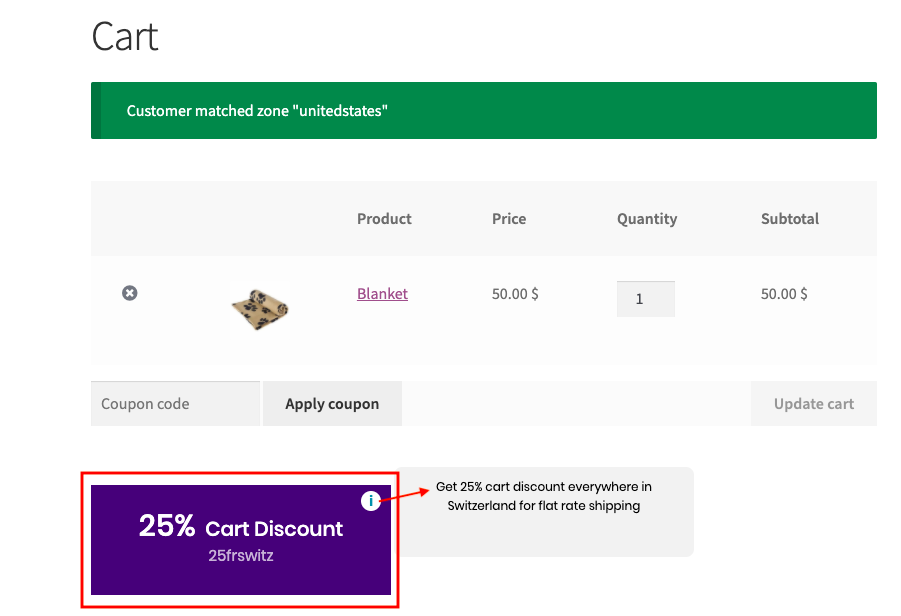This image features a detailed screenshot of the cart page from an online shopping website. In the top left corner, the word "Cart" is prominently displayed. Directly below, a green banner reads "Customer Match Zone" followed by "toUnitedStates" with no spaces and all in lowercase letters. 

The screenshot indicates that the user has added one item to their cart: a beige blanket adorned with black dog paw prints. This blanket is priced at $50. Below the blanket details, there is a section labeled "Coupon Code" with an adjacent button labeled "Apply Coupon." The coupon code box is currently empty. 

Additionally, an "Update Cart" button is visible but grayed out, rendering it non-selectable. Beneath this, a highlighted area announces a "25% Discount," accompanied by a coupon code "25FRSWITZ." An arrow extends from this code pointing to another box, which explains, "Get 25% cart discount everywhere in Switzerland for flat rate shipping."